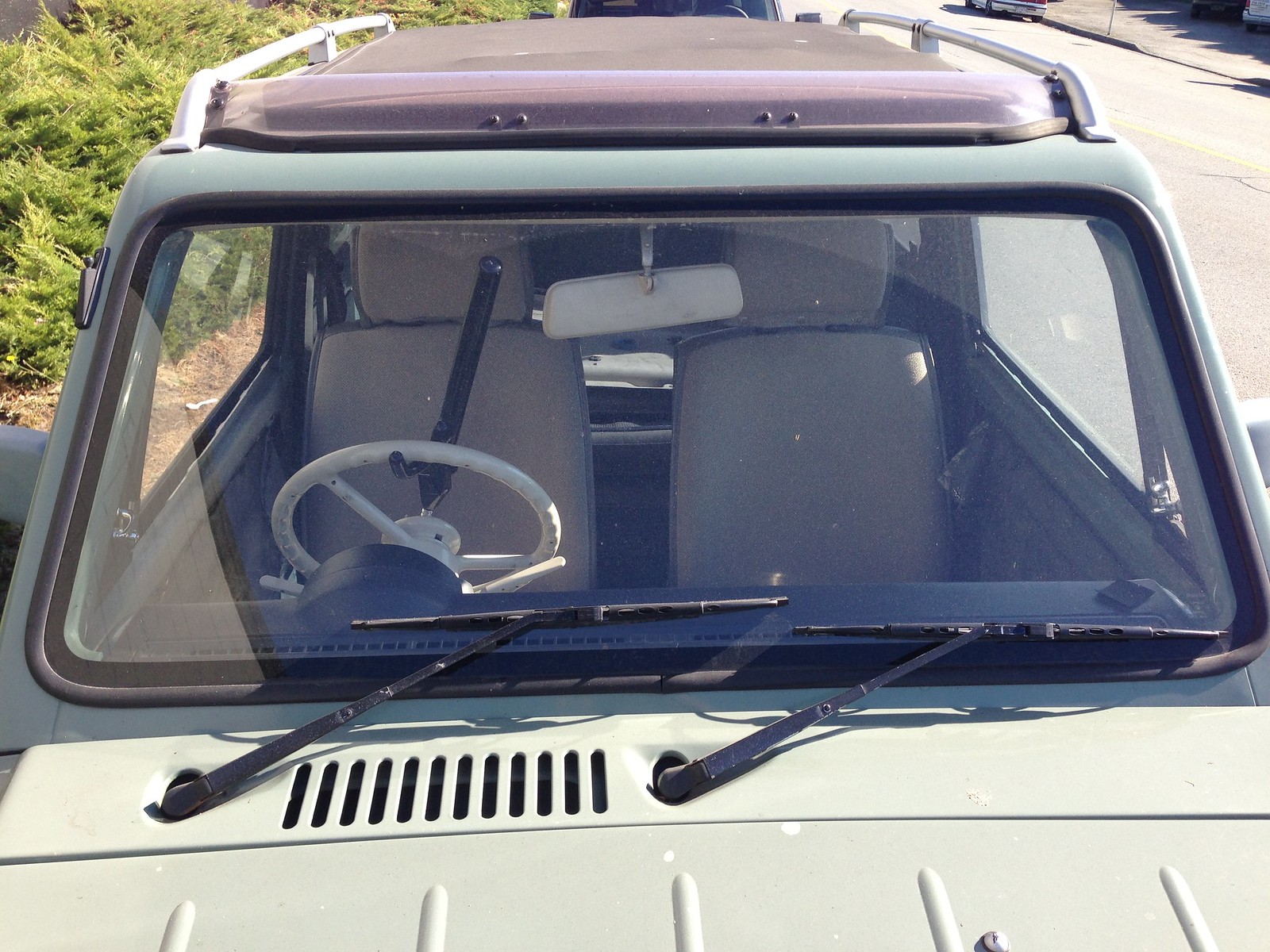This close-up photo captures the front of an old, light turquoise van or Land Rover on a sunny day. The image prominently features a rectangular, boxy windshield equipped with black wipers. The vehicle includes a tie rack on the roof and has all its windows shut. Through the clear windshield, you can see the right-hand drive interior, which features a white steering wheel secured with a theft-deterrent club device. The spacious, cloth bucket seats and absence of a center console suggest an older design. The background reveals lush green foliage and a bush to the right, along with a glimpse of a road.